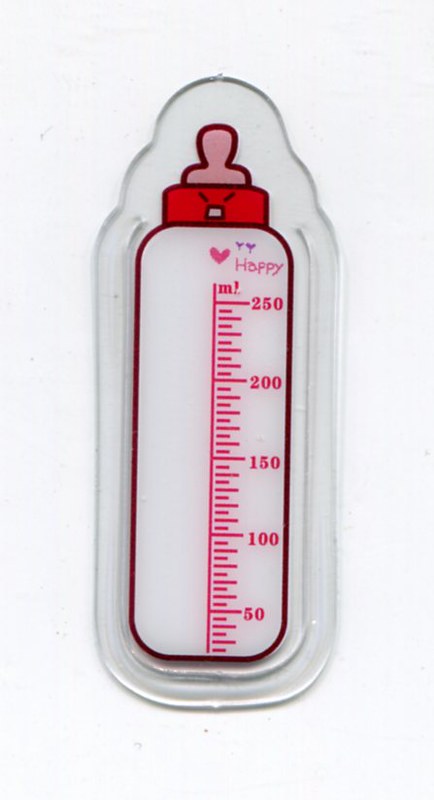In this meticulously detailed photograph, a baby bottle sits centrally atop a reflective piece of glass. The bottle itself is strikingly outlined in black, while its main body is completely white, creating a stark contrast that emphasizes its features. Red markings artfully denoting volume measurements adorn the bottle's exterior, starting from zero and ascending in precise 50 milliliter increments up to 250 milliliters. Between each primary 50 milliliter mark, the scale is finely segmented into smaller units, ensuring accurate measurements.

The bottle is capped with a vibrant red lid, which securely holds a pink-tinted nipple, highlighting the product's functional design. Intriguingly, the red cap features a small square emblem from which two line segments extend diagonally from each upper corner, forming a carefully considered 45-degree angle. The entire assembly is elegantly showcased against a similar glass background, producing a cohesive, sleek visual effect that emphasizes both form and function.